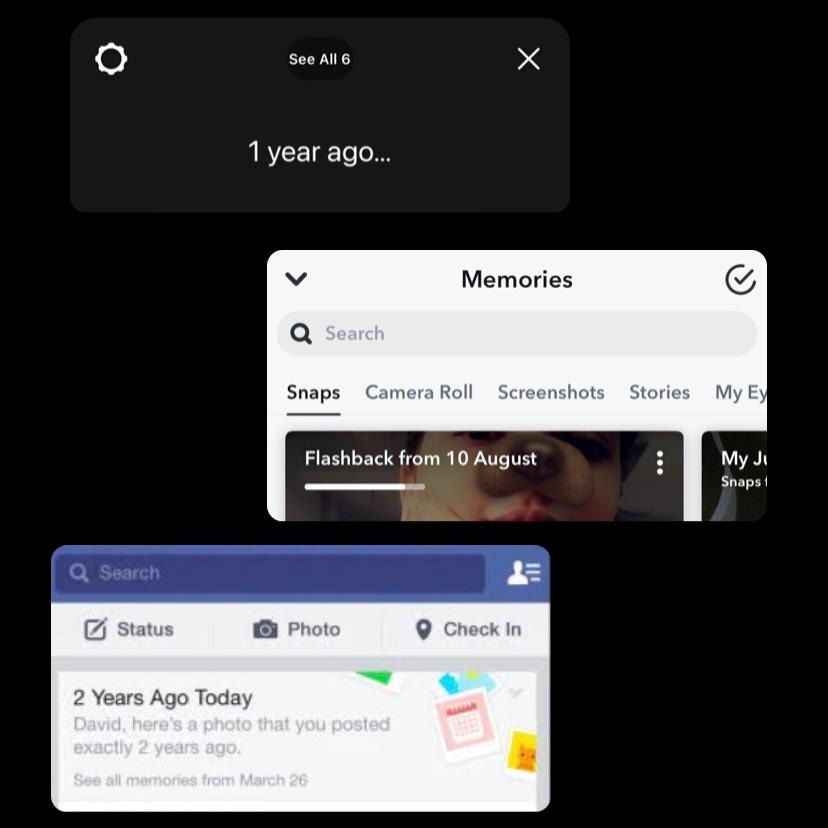This screenshot, set against a solid black background, features various interface elements and a partial image. 

In the upper left corner, there is a white settings icon. Adjacent to it, in small white text, are the words "See All," followed by a white "X" on the far right. Below these icons, in bold white text, is the phrase "One year ago…" 

Beneath this, a box has opened, displaying the word "Memories" against a white background. To the right of "Memories" is a checkmark, and to the left is a pull-down arrow. Directly below this, there is a gray search bar with 'Search' written in light gray text and accompanied by a magnifying glass icon.

Below the search bar, a horizontal menu stretches from left to right, including the categories: "Snaps" (which is highlighted and underlined as a link), "Camera Roll," "Screenshots," and "Stories." 

At the bottom of the screenshot, there is a partial view of a photo. The top of the photo is overlaid with the text "Flashback from 10 August." The visible portion of the image appears to show someone's head.